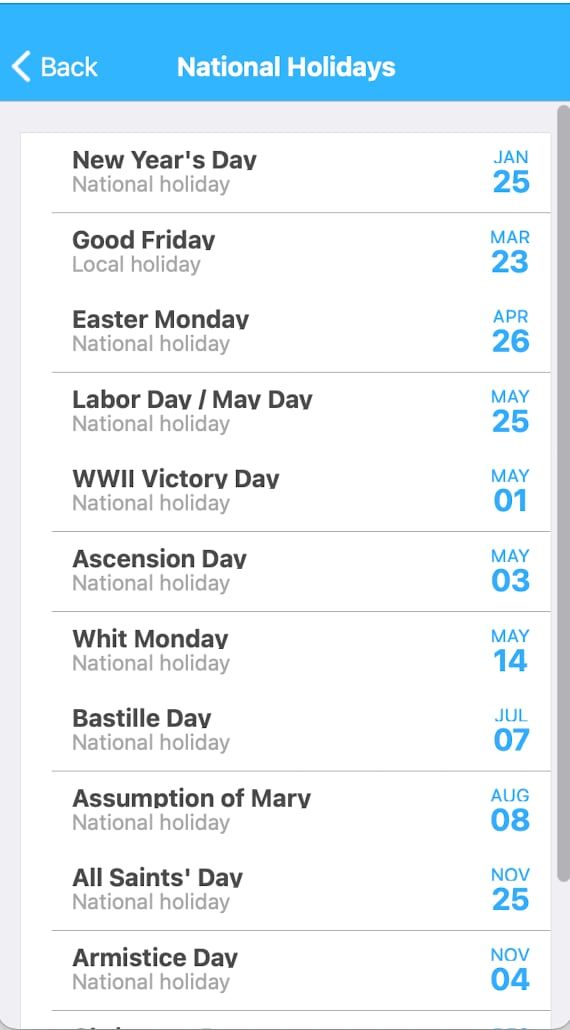The image depicts a mobile application displaying a list of national holidays. The app interface is designed to resemble a phone screen, complete with rectangular boxes listing each holiday. At the top of the screen, a blue bar features the label "National Holidays" in white text, alongside a white "Back" button.

The holiday list includes the following entries, each within its own box and separated by horizontal lines:
- New Year's Day: January 25th
- Good Friday: March 23rd
- Easter Monday: April 26th
- Labor Day (May Day): May 25th
- World War II Victory Day: May 1st
- Ascension Day: May 3rd
- Whit Monday: May 14th
- Bastille Day: July 7th
- Assumption of Mary: August 8th
- All Saints' Day: November 25th
- Armistice Day: November 4th

The holiday names are written in black text, with the dates highlighted in the same blue as the top bar. Beneath each holiday name, a gray subtitle indicates whether it is a national holiday. 

Based on the holiday dates and names, it is apparent that the app is not related to the United States, as New Year's Day is listed as January 25th instead of January 1st.